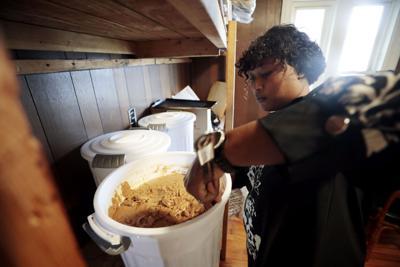The image features a woman with short black, curly hair and a black and white short-sleeve t-shirt, standing in what appears to be a rustic kitchen or shed-like interior. She is reaching her left hand into a deep, white pot with black handles, possibly cooking or preparing food. In the background, to the right, there is a dual-paned window or door with a white frame, adding natural light to the space. The setting is detailed with wooden walls and flooring, as well as a wooden shelving unit on the left and a wooden beam visible. Below the wooden shelf, there are two additional white containers, likely used for food storage, that are sealed. A power outlet is situated in the center of the wooden counter, indicating a functional cooking or prep area. The overall scene provides a cozy, intimate glimpse into a perhaps smaller, well-utilized kitchen space.